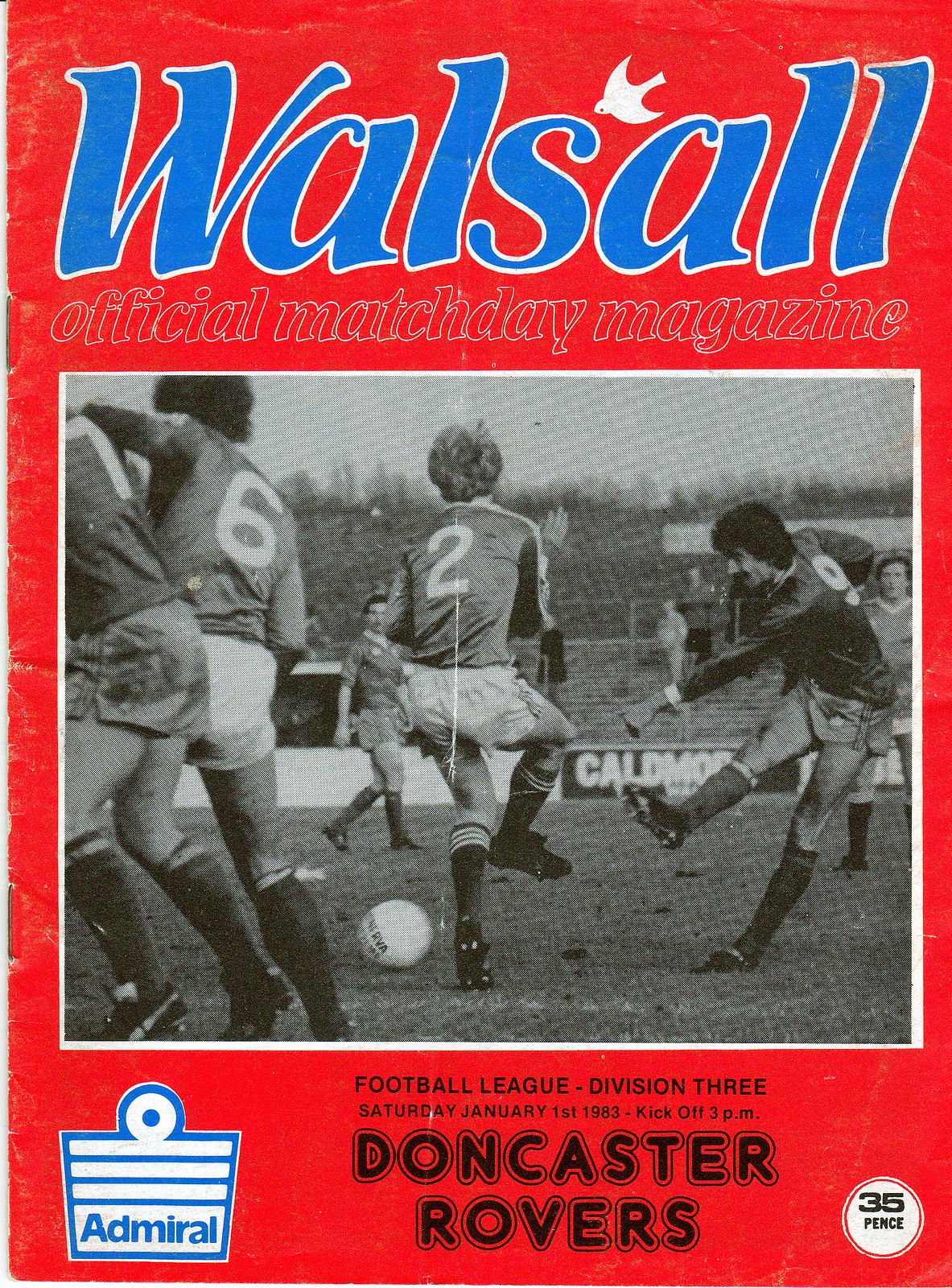The cover of this vintage Official Matchday Magazine boasts a bold red background with the title "Walsall" in large, bright blue letters with white borders prominently displayed at the top. Nestled between the letters "S" and "A" is a distinctive white bird emblem. Positioned just beneath the title are the words "Official Matchday Magazine" in red font outlined in white. Occupying the central section is a black-and-white photograph showcasing a lively soccer match. In this image, players donning light shorts and dark socks are in action, with visible jersey numbers such as 7, 6, and 2. The scene includes a white football on the grass, with players engaging intensely around it. The background of the photograph reveals sparse audience stands, a hill adorned with trees, and an expansive sky. Alongside the field, sponsor advertisements such as "Calmon" are visible. In the bottom left corner of the cover, a logo resembling a white can or pail with blue detailing and the word "Admiral" inscribed in blue is present. Below the central image, black text details the event: "Football League, Division III, Saturday, January 1, 1983, kickoff 3 p.m., Doncaster Rovers." Finally, in the bottom right corner, a small white circle displays the price, "35 pence," in black font.